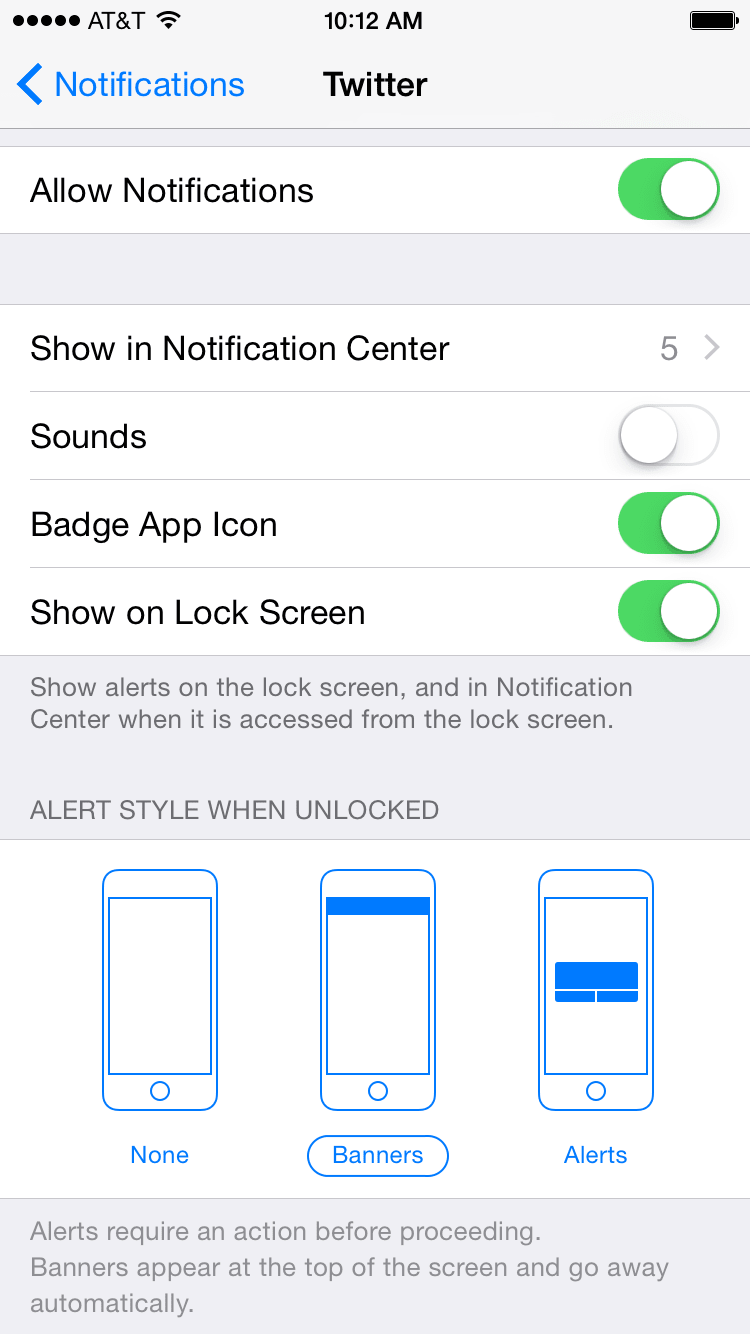Here is the cleaned-up and detailed caption:

---

This image is a screenshot of a smartphone displaying notification settings for the Twitter app. 

In the upper left-hand corner, the status bar shows an AT&T logo next to a Wi-Fi signal indicator with five black dots. Centrally positioned at the top, the time is displayed as 10:12 AM. In the upper right-hand corner, there is a full battery icon.

Directly below the status bar, there is a blue left-pointing caret symbol followed by the word "Notifications" in blue text. To the right, the title "Twitter" is centered.

The page contains several toggle switch options for configuring Twitter notifications. The first option, "Allow Notifications," is enabled, indicated by a green slider button. Below this, a gray divider bar separates the next setting. The second option, "Show in Notification Center," includes a light gray number '5' and a right-pointing caret symbol.

Following this, the "Sounds" setting is listed with its toggle switch turned off. The "Badge App Icon" option is next, with its associated switch currently turned on. The "Show on Lock Screen" setting follows, also enabled.

A gray rectangular text box beneath these options reads: "Show alerts on the lock screen and in Notification Center when it is accessed from the lock screen." Finally, the "Alert Style When Unlocked" section shows three diagram options—None, Banners, and Alerts—for configuring the visual alert style when the device is unlocked.

---

This caption provides a descriptive and organized overview of the screenshot, outlining the relevant details and layout of the notification settings interface for the Twitter app.